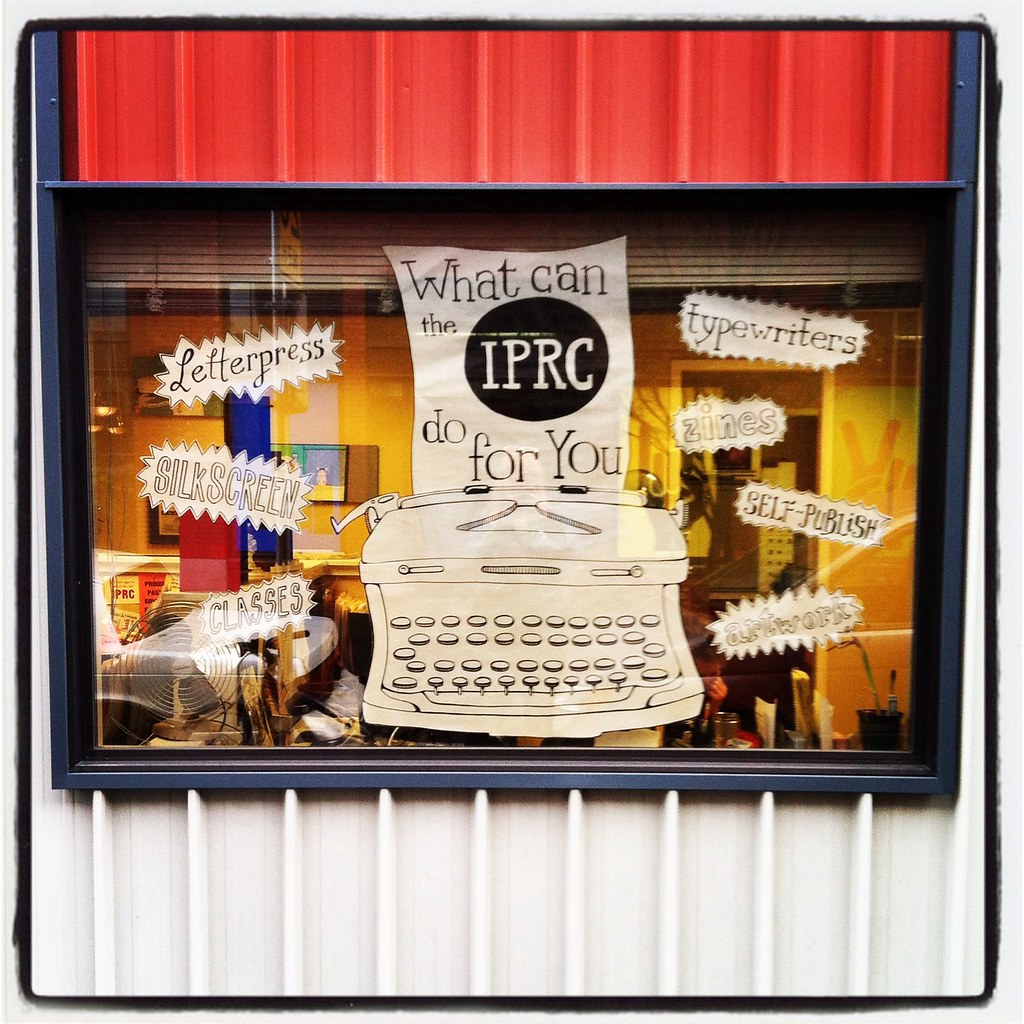In this image, a white corrugated metal wall serves as the background, with a window framed in blue metal at its center. The upper part of the wall is red, while the lower part is off-white. Inside the window, various decals are displayed, the most prominent being a black typewriter with off-white paper. The paper bears the text: "What can the IPRC do for you?" in black print, with the acronym "IPRC" highlighted in a black circle with white lettering.

Surrounding the typewriter, speech bubble decals list activities and services: "letterpress," "silkscreen," "classes," "typewriter," "zine," "self-publish," and "artwork." Through the window, you can see a classroom with bright yellow walls, desks adorned with pencils and letters, and a fan. A person appears to be working inside. This detailed setup likely serves as an advertisement for the various creative resources and classes offered by the IPRC.